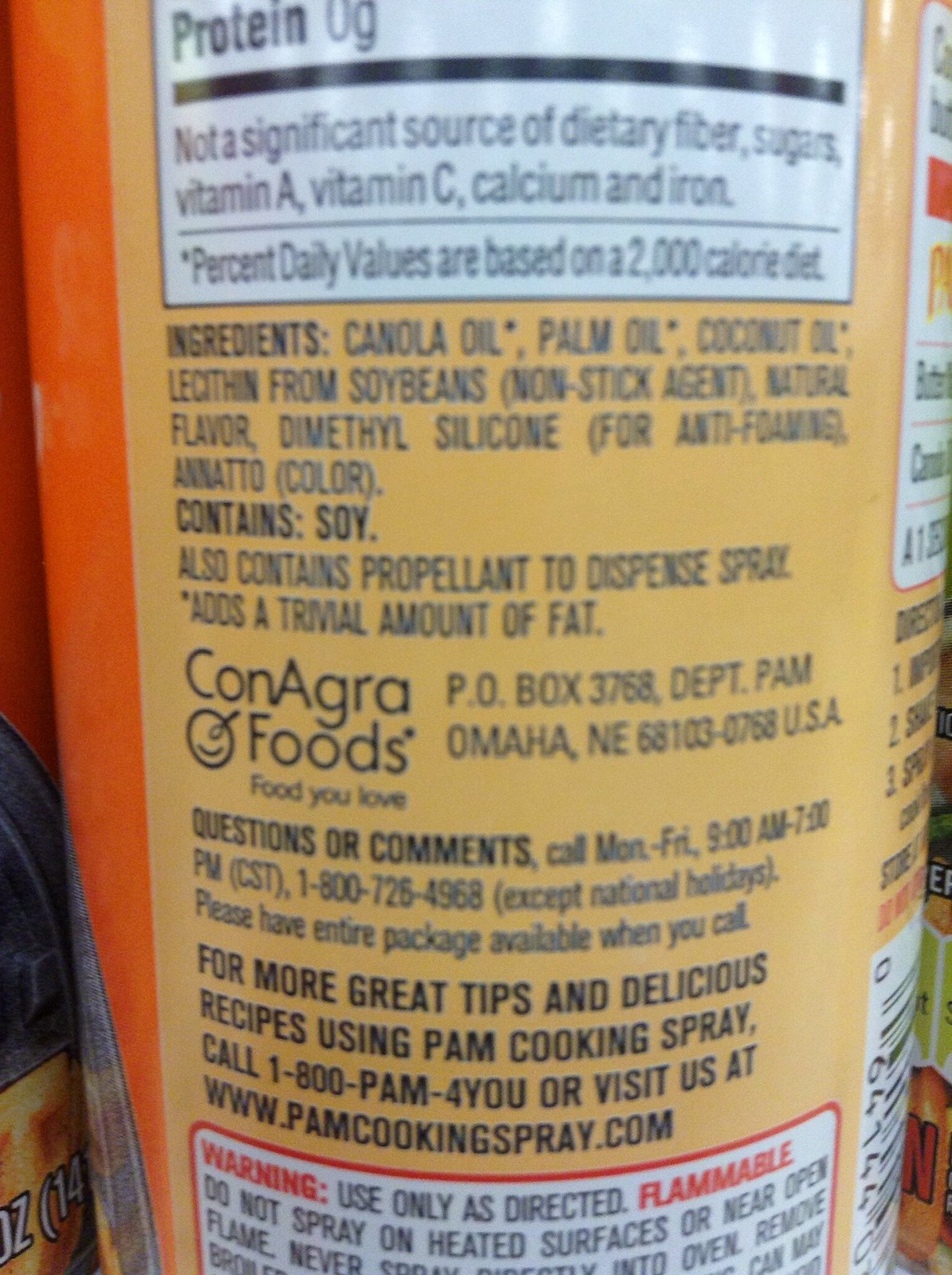This image displays a cylindrical container, positioned to show the detailed label on its backside. The label is segmented into three distinct sections. The top and bottom sections are bordered by black rectangles and feature a stark white background with black text. At the top, nutritional information highlights that the product contains zero grams of protein and is not a significant source of dietary fiber. 

The middle section, set against a yellow-brown background, lists the product's ingredients and manufacturing information. The ingredients include canola oil, palm oil, coconut oil, lecithin derived from soybeans, a nonstick agent, natural flavor, dimethyl silicone for anti-foaming, and annatto for color. It notes that the product contains soy and utilizes a propellant for dispensing the spray, which adds a trivial amount of fat. 

Based on the description, this is a type of nonstick cooking spray intended for use on cooking utensils. The product is manufactured by ConAgra Foods, based in Omaha, Nebraska.